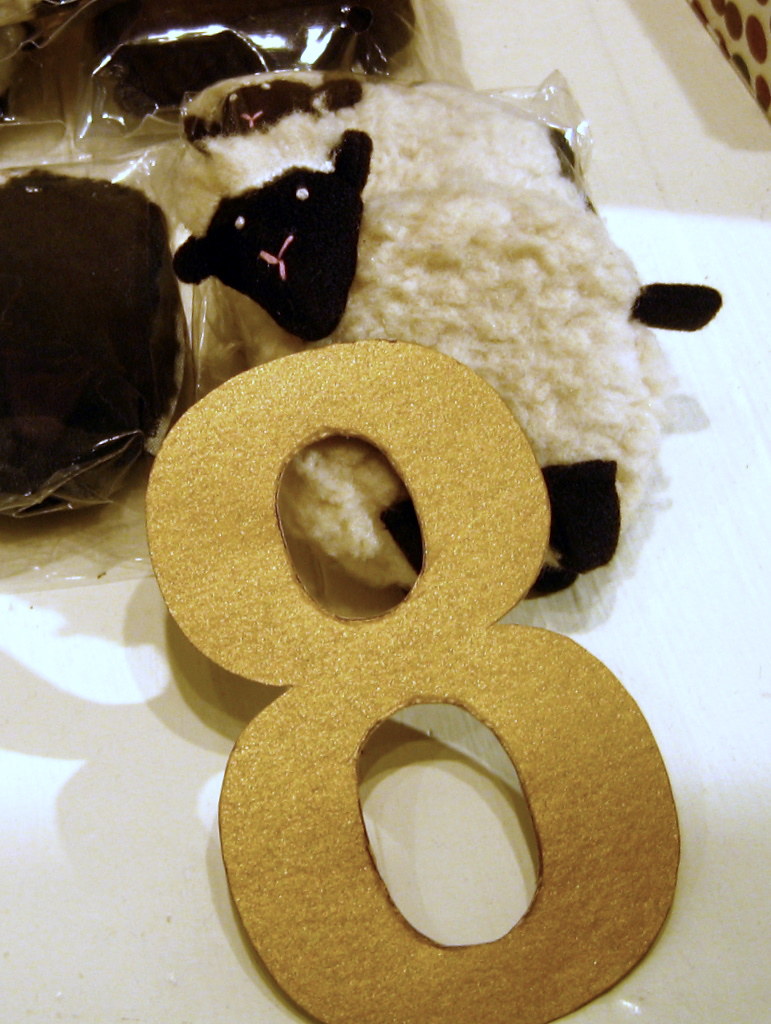The photograph features two plush sheep toys adorned with bushy white fur, black feet, and black faces each with a distinctive red nose. These whimsical sheep are seated on a pristine white table, slightly overlapping with a large, glittery gold number eight—likely made from cardboard—resting atop them. This gold numeral, probably intended as a decorative item for celebrations, casts a shadow toward the left of the frame due to a light source originating from the top right. Just behind the sheep and to their left is a small, round black object wrapped in plastic, possibly a makeup bag or case for electrical items. The entire scene is bathed in a soft light, enhancing the playful yet detailed composition.